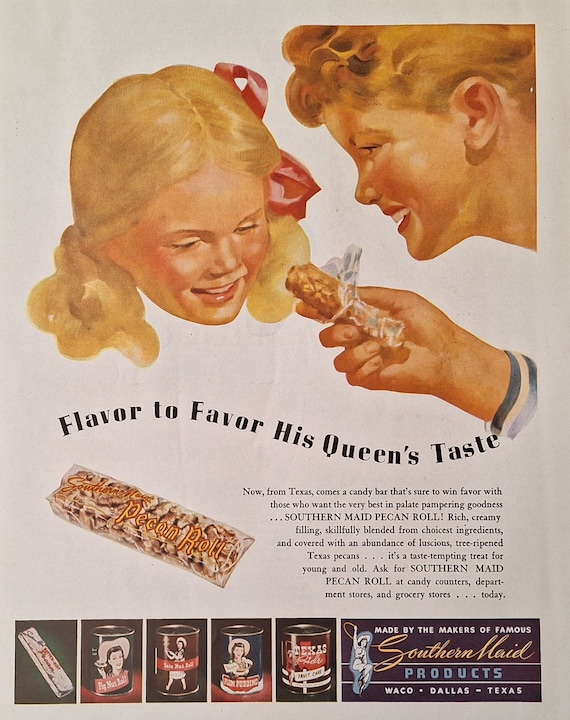In this vintage advertisement, likely from the 1940s or 50s, we see a charming, painted scene with a light blue background. Dominating the image is a young girl with blonde hair styled in pigtails adorned with a red ribbon, joyfully smiling with rosy cheeks. To her upper right, an older woman with reddish-blonde hair, also smiling, is offering her a candy bar. The woman's hand is visible, holding the unwrapped, brown pecan roll. Below this heartwarming interaction, the curved tagline reads, "Flavor to Favor, His Queen's Taste."

To the left below this tagline, there is a visual of the pecan roll in its packaging, marked with "Southern-made Pecan Roll" in prominent lettering. Adjacent to this, to the right, is a descriptive paragraph detailing the candy's rich, creamy filling and abundance of luscious, ripe Texas pecans, promising a taste-tempting treat for both young and old. Splashed across the bottom of the ad are smaller images of the brand's other products, including a bar, a square item, and four cans featuring a girl with a cowboy hat in the middle, all tagged with the phrase "Made by the makers of famous Southern-made products, Waco, Dallas, Texas."